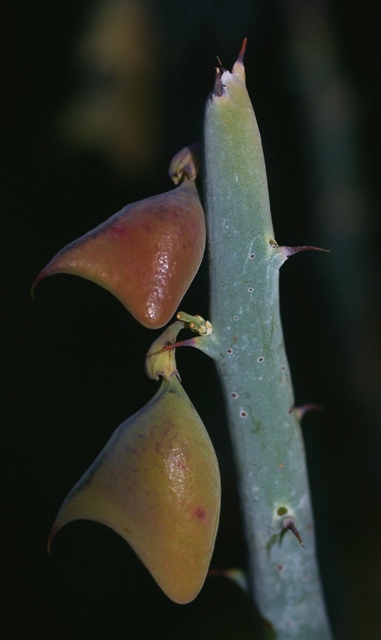This close-up image captures the top of a distinctive, cactus-like plant against a dark, blurry background. The main stalk is green with a waxy texture, adorned with red spikes that jut out sharply. The plant features small, triangular buds that resemble either flower buds or seed pods. The uppermost bud has a brownish-red hue, while the larger, lower one is green with red speckles, its shiny surface evoking that of fruit. Alongside the spikes, there are two prominent leaves on the left side that curve gracefully. These leaves transition in color from a darker brown at the top to a lighter brown towards the bottom and exhibit a waxy texture. The plant’s surface also displays scattered dots, possibly pores. In the dim background, subtle white highlights can be noticed, enhancing the plant's vivid green and red detailing.